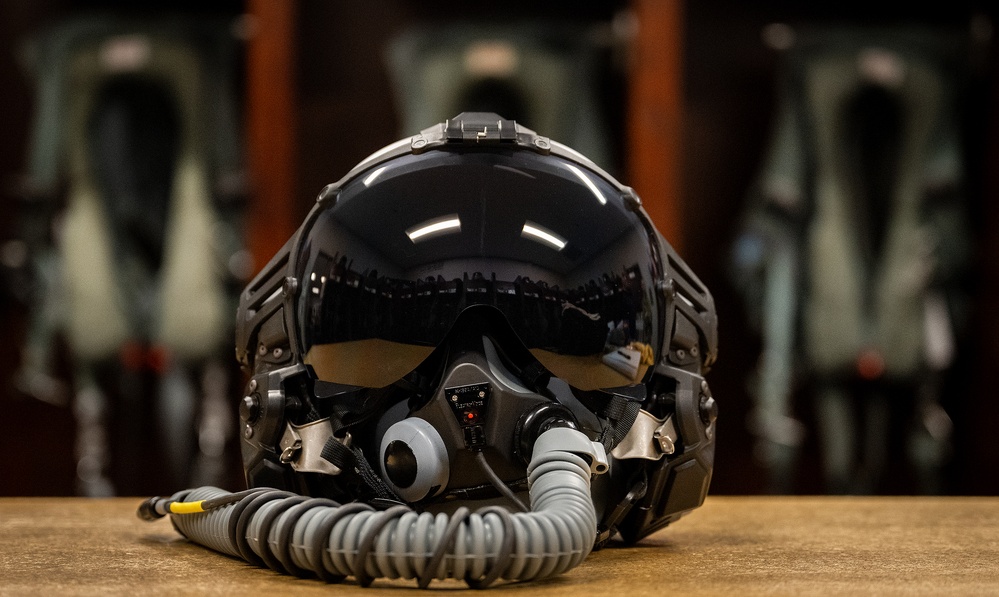This photograph features a detailed image of a black flight helmet, resting on a medium-colored wooden table. The helmet is equipped with a full eye-covering shield, which appears almost black or tan see-through, designed to protect the wearer's eyes from sunlight. The helmet showcases various rivets and straps, adding to its rugged appearance. A prominent feature is the mouthpiece, which includes a triangular apparatus with an illuminated light at the very center. On the left side of the mouthpiece, there's a respirator valve, and a long, light gray oxygen tube extends from this area, wrapped in a dark gray cord.

In the background, three blurry suits can be seen, possibly indicative of uniforms or gear for activities like paintball or laser tag. These suits are arranged with a red wooden wall as their backdrop, and they appear to be in shades of gray, white, and black. The intricate details of the helmet and its supplementary equipment suggest its use in aviation or similar high-intensity environments.